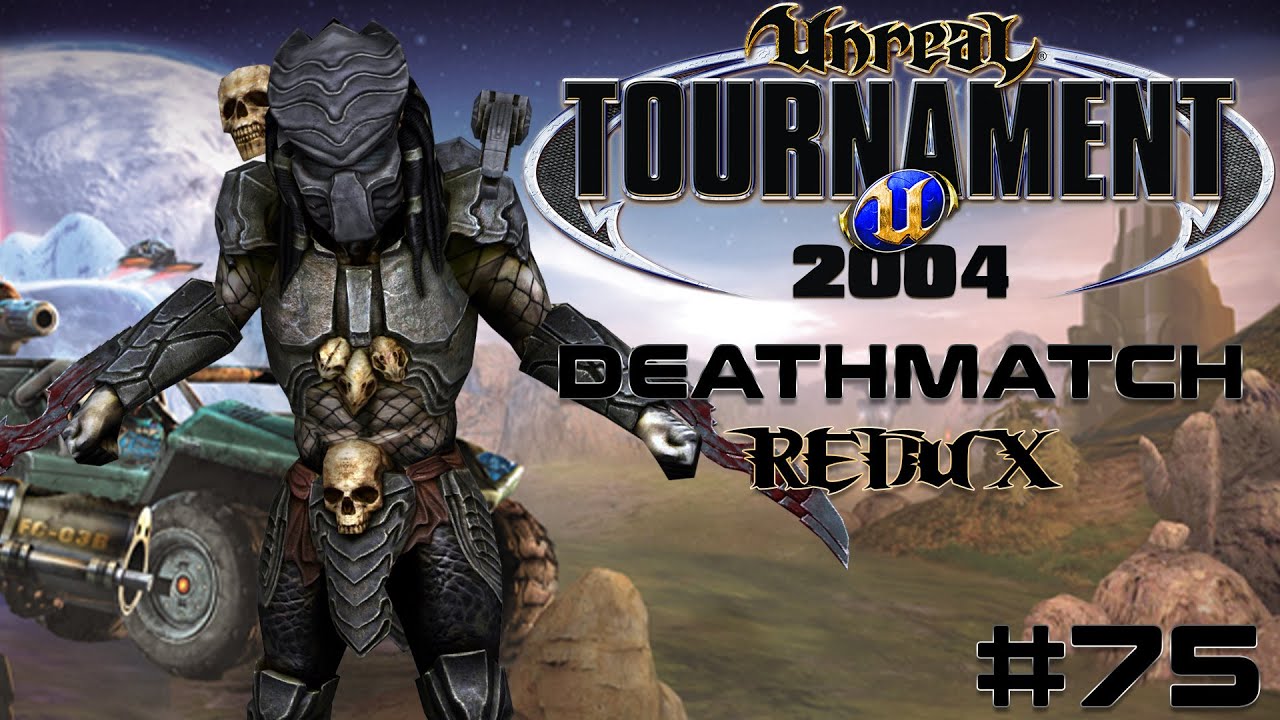This is a computer-generated advertisement poster with a black background featuring a prominently placed logo in the upper right corner. The logo consists of the word "UNREAL" in huge white letters followed by "TOURNAMENT" and then the year "2004." Below, in thinner large letters, it reads "DEATHMATCH" and "Redux." At the bottom right, the number "75" is displayed in large font. On the left side of the poster stands a menacing, alien-like character reminiscent of the Predator from the renowned movie franchise. This character is dressed all in black combat gear with a hard black mask, wearing a skull as a belt buckle. The character has its arms open, wielding a knife in its left hand. Behind it stands a jeep-like vehicle, suggesting a battleground setting. Further in the background, a desert landscape and a rising moon or planet are visible, enhancing the eerie and otherworldly atmosphere of the poster.